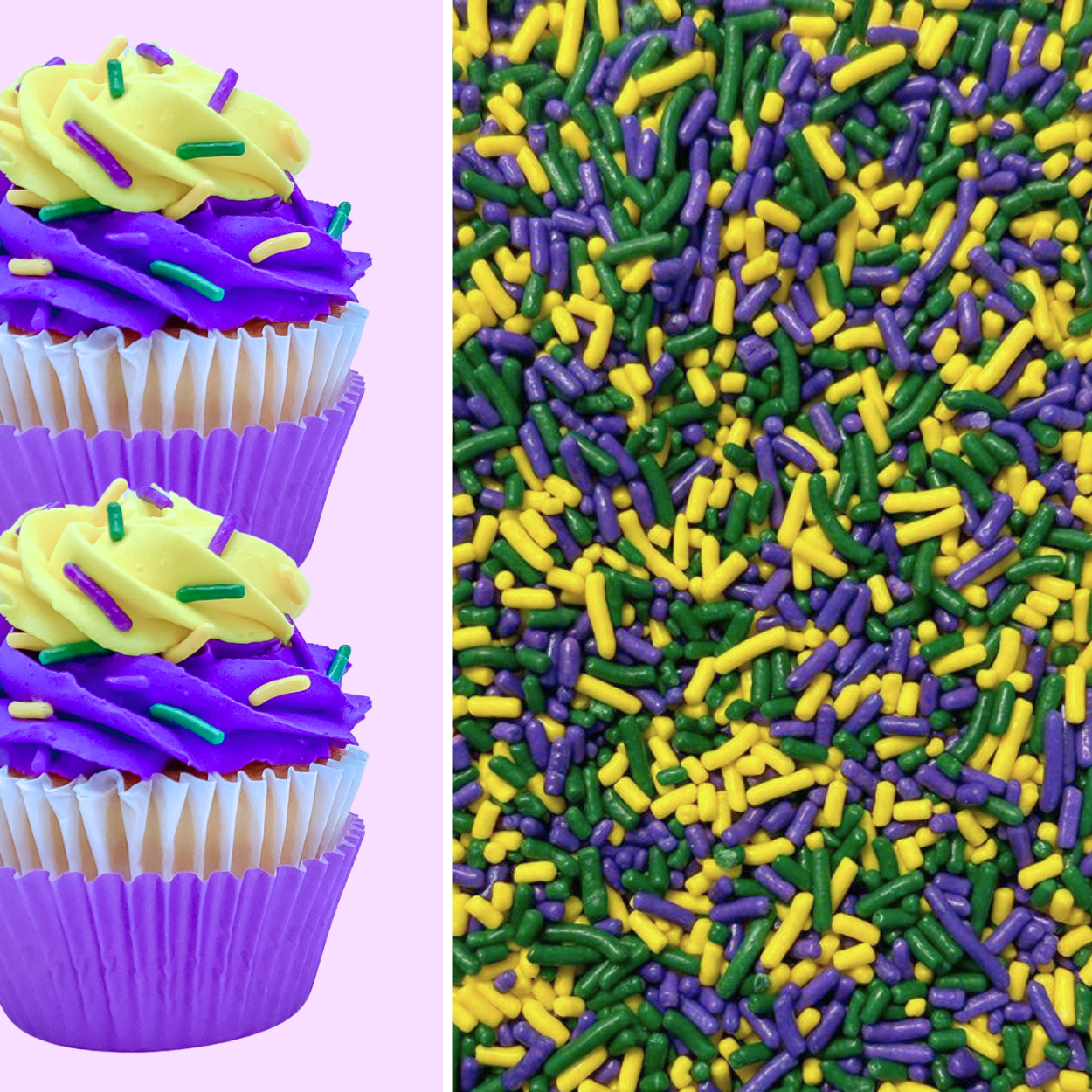The photograph is divided into two parts, with the left third displaying two identical cupcakes and the right two-thirds featuring a dense spread of colorful sprinkles. The cupcakes are positioned on a pale pink background and are stacked vertically. Each cupcake is encased in two wrappers - an outer purple cup and an inner white lining. The cake portion, likely red velvet, peeks out above the white liner. Topped with a swirl of purple icing and a dollop of yellow icing, the cupcakes are adorned with vibrant sprinkles in hues of purple, green, and blue. The right side of the image showcases a close-up of the same sprinkles, filling the entire space with their green, yellow, and purple colors. The overall theme of the image, emphasized by the repeated colors and elements, appears to be centered around a bright and festive palette, predominantly featuring purple.